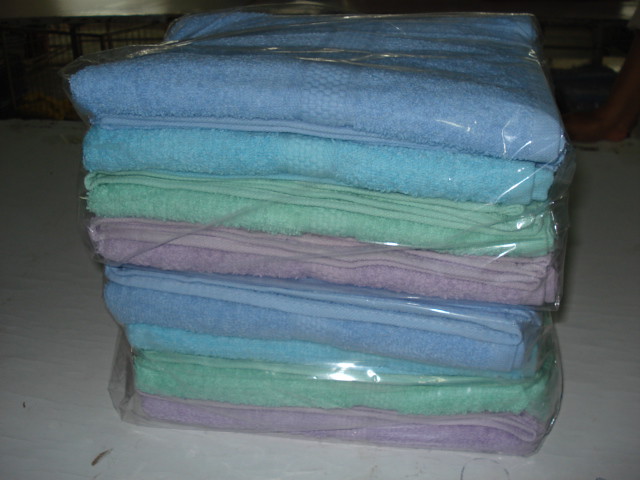This image shows a detailed scene featuring a stack of brand new, neatly folded towels encased in plastic bags. The towels are arranged on top of each other, each set contained within its own plastic wrapping. They are placed on a white surface, which could be a table or bedding, adding a clean background to their presentation. The two towel sets are identical, with each set consisting of four towels stacked in the same consistent pattern: a light purple towel on top, followed by a light blue towel, a teal green towel, a darker blue towel, and a light pinkish purple towel. This sequence is repeated in the second set, creating a visually balanced arrangement of eight towels in total. Each towel has a textured detail running along its shorter edge. The setting also includes a gray floor that might be hardwood or vinyl, though the background remains blurred, keeping the focus solely on the colorful and neatly packaged towels.